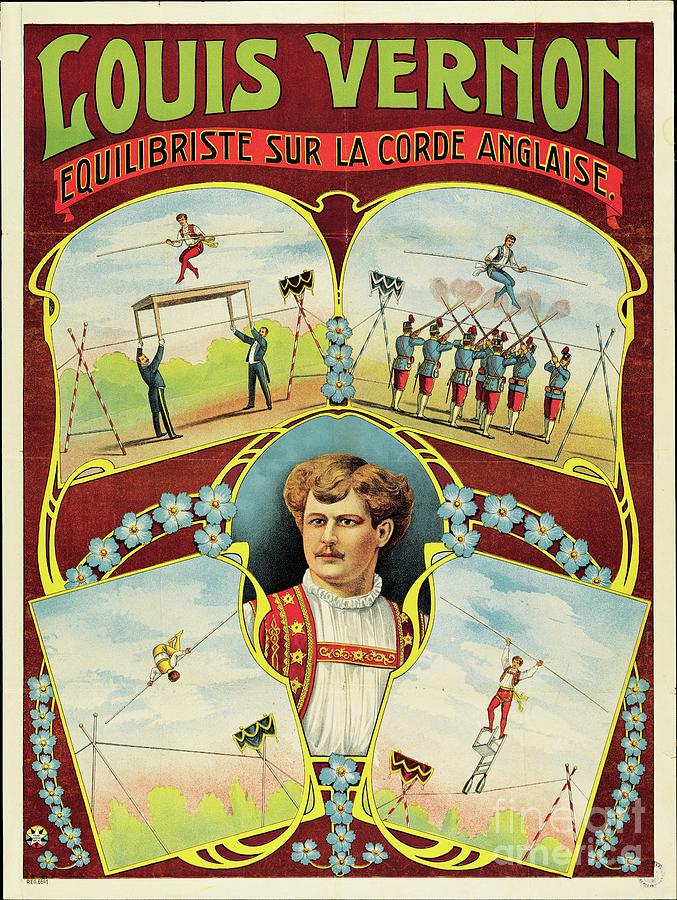This vividly colorful poster advertises the circus performer Louis Vernon, prominently featured at the top in green letters against a maroon background. A rectangular red banner with black letters below his name reads "Equilibrist sur l'Accord Anglaise," indicating his specialty in balancing acts. Centrally, a drawing of Louis Vernon himself captures attention, depicting him with wavy brown hair, a mustache, and dressed in a distinctive white ruffled shirt and red vest secured by a strap. Surrounding him is a series of intricate, detailed drawings showcasing various acrobatic feats: two men holding up a table as Vernon balances across it with a rod; another scene of him walking across criss-crossed guns held by men; and an image of Vernon balancing precariously on an upside-down chair atop a wire. The border of this elaborate composition is white, adorned with blue flowers that enhance the visual appeal. This poster effectively highlights both Vernon's impressive balancing skills and his charismatic stage presence, likely aimed at promoting his circus acts.